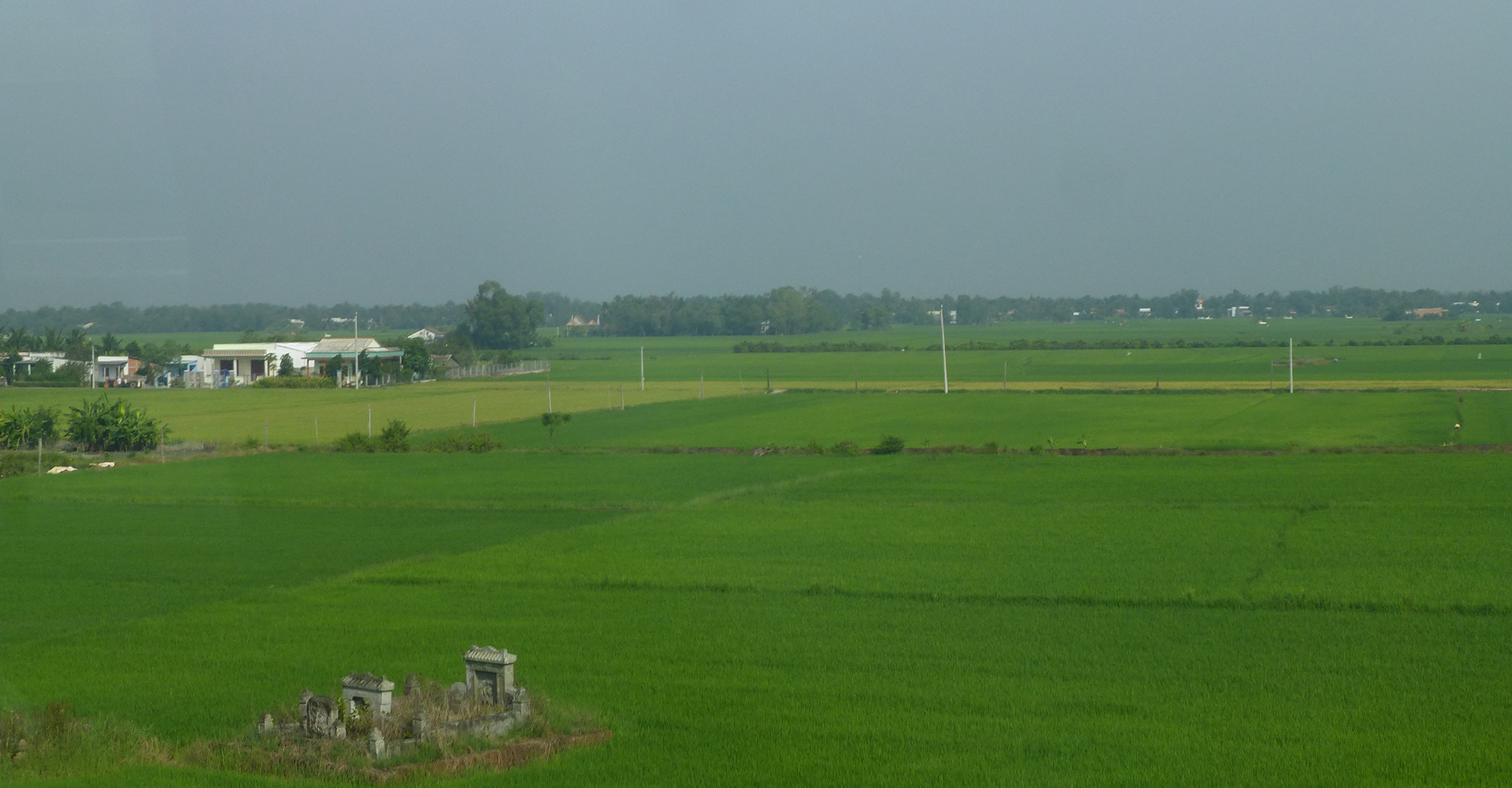A sprawling landscape photo captures a lush green field stretching far into the distance under an overcast, gray sky. The field is thriving with vegetation, possibly crops, amidst patches of overgrown brush and some bushes. In the foreground, white electrical poles stand tall, marking the terrain. To the left and center of the image, there are remnants of stone structures, possibly a mausoleum or old ruins, hinting at a small, overgrown graveyard or the remains of a house. A modern building complex, mainly white, can be seen towards the top left, with a haze of more structures and potential roadways just visible on the horizon. The horizon is framed by a line of distant trees, completing the serene yet slightly somber scene. The overall atmosphere suggests that it could be raining, adding to the melancholic tone.